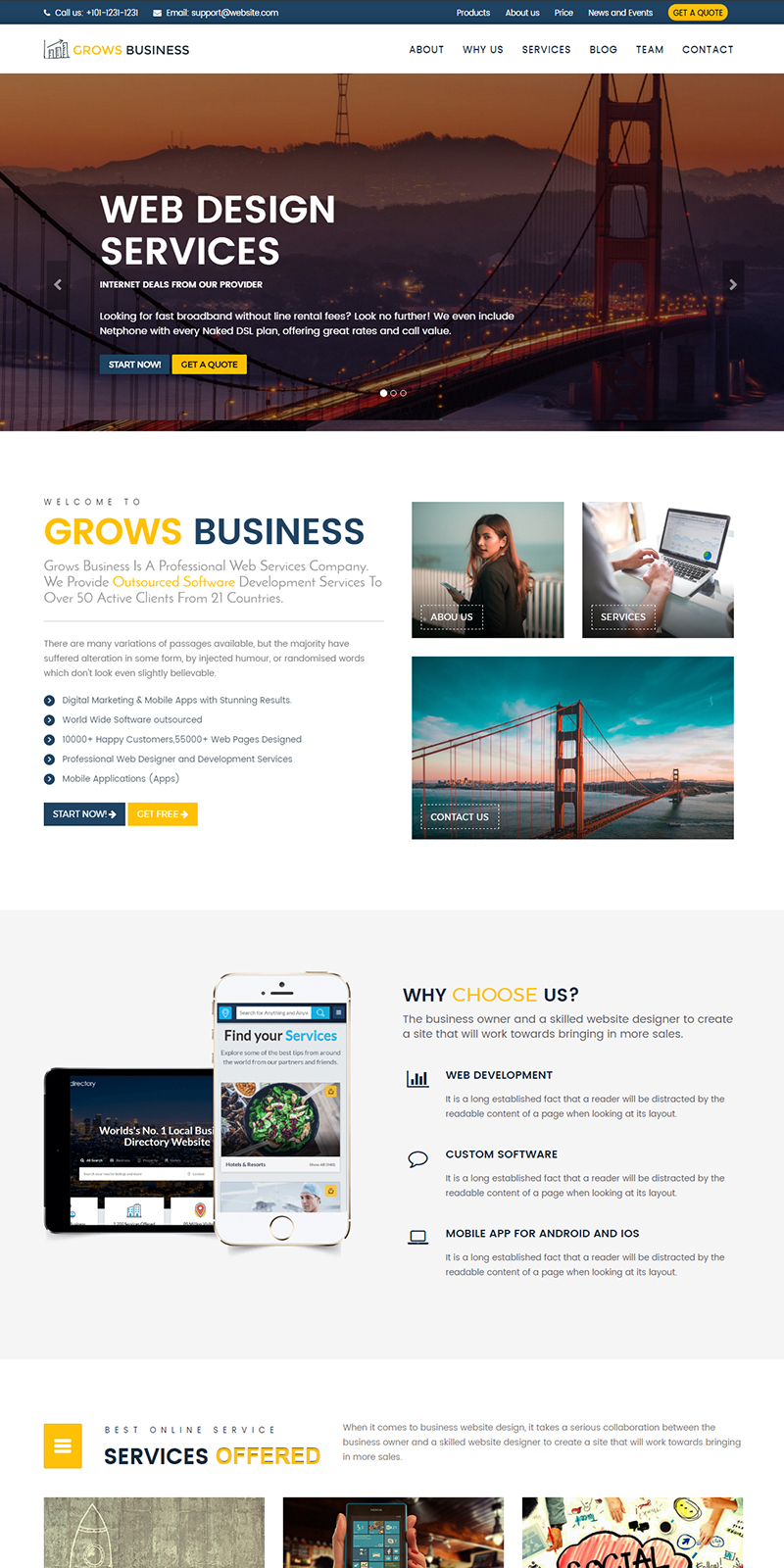A screenshot of a business website showcasing web design services. At the top, a small blue banner features a menu, followed by an inch-wide white banner with yellow text. Accompanying, smaller blue text reads "business," but its full content is unreadable due to the screenshot's size. 

Below, a background image of the Golden Gate Bridge highlights the section headlined in bold white text: "Web Design Services." Beneath this, the background transitions to white, with yellow text reading "grows" and adjacent blue text stating "businesses." 

To the right, there are three images: one of a person, another of someone typing on a laptop, and lastly, an image of the Golden Gate Bridge again. 

Further down, below the "grows businesses," there's a wall of text too small to read. The background then shifts to gray, showcasing an image of a tablet and a phone displaying web design service examples, overlain with the phrase "Why Choose Us." This section includes unreadable supporting text and three bullet points.

At the bottom, labeled "Services Offered," there is another paragraph of text, with three partially visible images beneath it. Although much of the text is too small to read, the overall layout comprehensively presents the company's web design services.